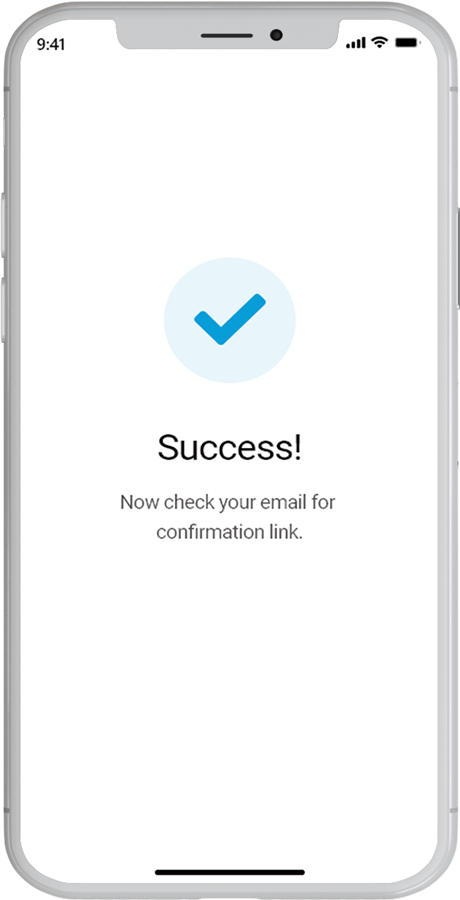This is a meticulously detailed illustration of a standard-size cell phone, positioned to face the viewer directly. The phone features a light gray rim encircling the entire device. The background surrounding the phone is predominantly white, complemented by a near-purely white screen in the center.

Central to the image, slightly above the midpoint, is a light blue circle with no border. Within this circle, a thick, medium blue checkmark is prominently displayed. Positioned beneath the circle, in black font, is the word "Success!" followed by an exclamation mark. Below this, there are two lines of smaller black text that read: "Now check your email for confirmation link." The phrase "confirmation link" occupies its own line, right-aligned with the text above it.

Notably, the image features a considerable amount of empty white space below the text. Near the bottom, aligned with the lower middle section of the phone, there is a thick black line spanning roughly 40% of the phone's width, situated just above the light gray or silver border.

At the top of the phone's display, the time "9:41" is shown in black font in the upper left corner. Adjacent to this, the top rim dips down, forming a small horizontal area that includes another horizontal line across it, occupying approximately 15% of the image's height. In the upper right corner, three standard cell phone icons are displayed: a full horizontal battery, a full Wi-Fi symbol represented by three semicircles, and four ascending bars denoting full cellular signal strength.

The detailed elements and the clean layout create a clear and organized visual message, punctuated by the success notification and confirmation instructions.